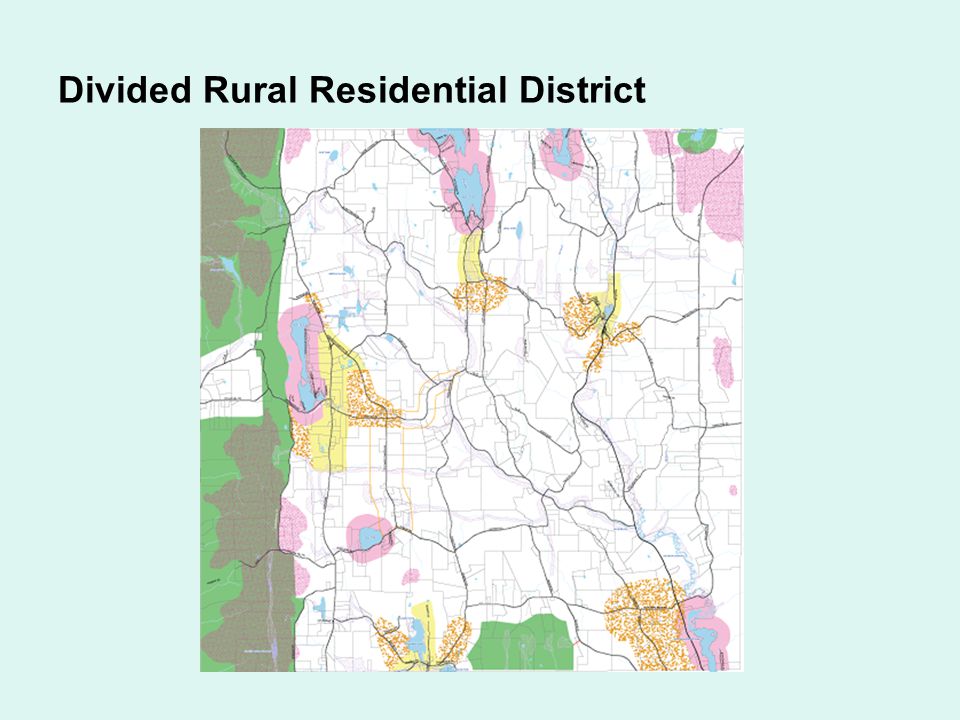This is an image of a graphic map set against a light blue background, depicting a "Divided Rural Residential District" as indicated by the black text title positioned near the top-left. The map itself is mostly white with splotches of pink, green, and blue. The blue areas likely represent bodies of water such as lakes and rivers, while the green indicates grassy or forested regions. Dark gray lines crisscross the map, illustrating the roadways that connect different parts of the district. Yellow shapes appear in certain areas, potentially signifying residential zones. The map also features some pink and orange or red areas, speculated to mark populated or potentially urban regions. Some parts of the map have a camouflage-like stripe, suggesting forested and unpopulated land. The whole image is surrounded by a thick lime border, emphasizing the district boundaries and adding to the map’s colorful detail.